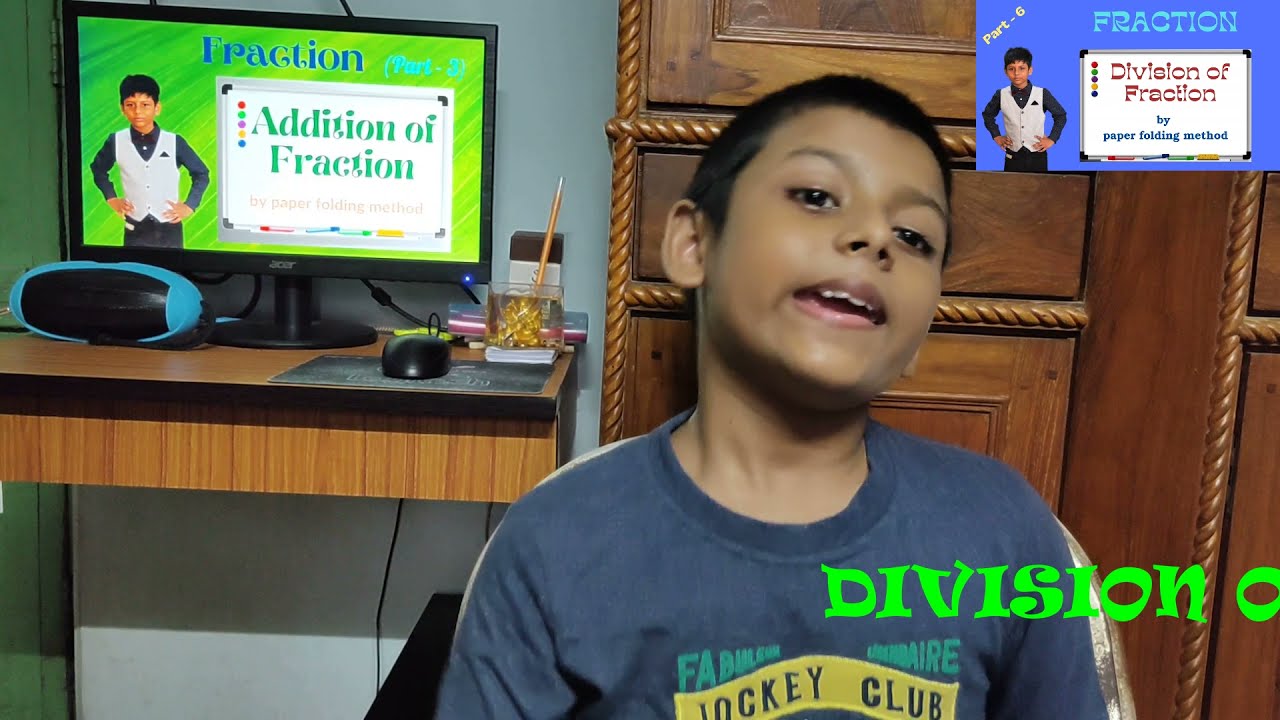In this horizontal rectangular image, a young boy is positioned on the right side, wearing a blue t-shirt that reads "Jockey Club" emblazoned in a yellow banner across the front. The boy, who has short dark hair, appears to be speaking directly to the camera while standing in front of a workspace that includes wood-colored office furniture—a desk with drawers visible behind him. On the desk sits a turquoise speaker, a computer monitor, and a scattering of various items like a mouse and pencil.

The computer screen, situated on the left side of the image, displays an educational interface. The background of the monitor is green, and prominently features a white box stating "Addition of Fraction." Above that, blue text reads "Fraction Part 3". In the upper left corner of the screen, there is another section highlighted in blue text saying "Fraction," with a white rectangle inside it reading "Division of Fraction." Notably, the same boy appears on the screen, now wearing a white vest over a dark blue shirt, with his hands on his hips, indicating a split-screen or multiple scenes in the video.

The top right corner of the overall image contains another blue square featuring the text "Fraction Part 6" and "Division of Fraction by Paper Folding Method." This pedagogical theme suggests that the boy might be part of an instructional video on mathematics.